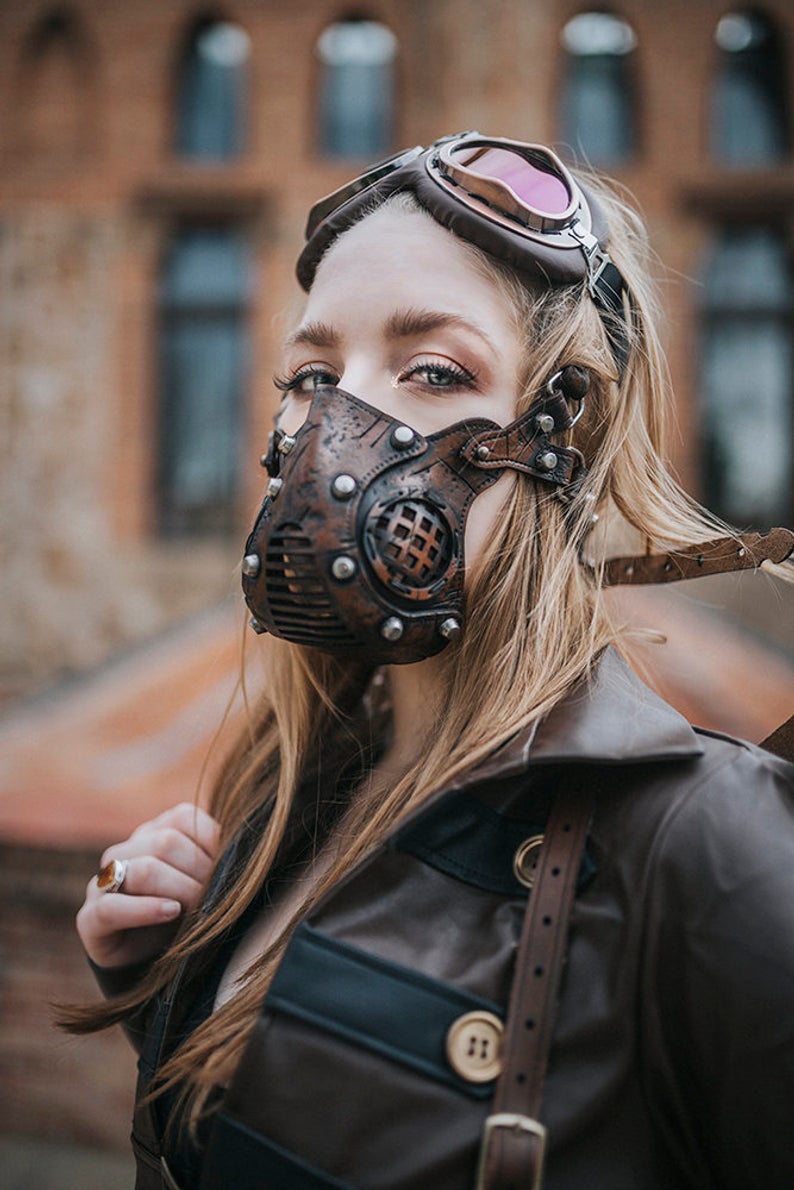In this close-up photograph, we see a young Caucasian woman with fair skin and striking blue eyes. Her long, honey blonde hair is styled straight and has darker roots near the scalp, transitioning to a lighter blonde towards the ends. She is wearing a distinctive steampunk-style gas mask made of solid, dark brown leather, adorned with large silver rivets. The mask, giving off a heavy and robust appearance, is fastened at the back of her head with a belt-like fastener. Positioned as a headband on her head, the brown leather-rimmed goggles complement the mask, adding to her steampunk aesthetic. She is dressed in a brown leather jacket that features black bands and holds the strap of a bag over her left shoulder with her right hand, which has an amber-like ring on one of her fingers. The background reveals a blurred, tall brick building with high and narrow windows, suggesting an urban setting.